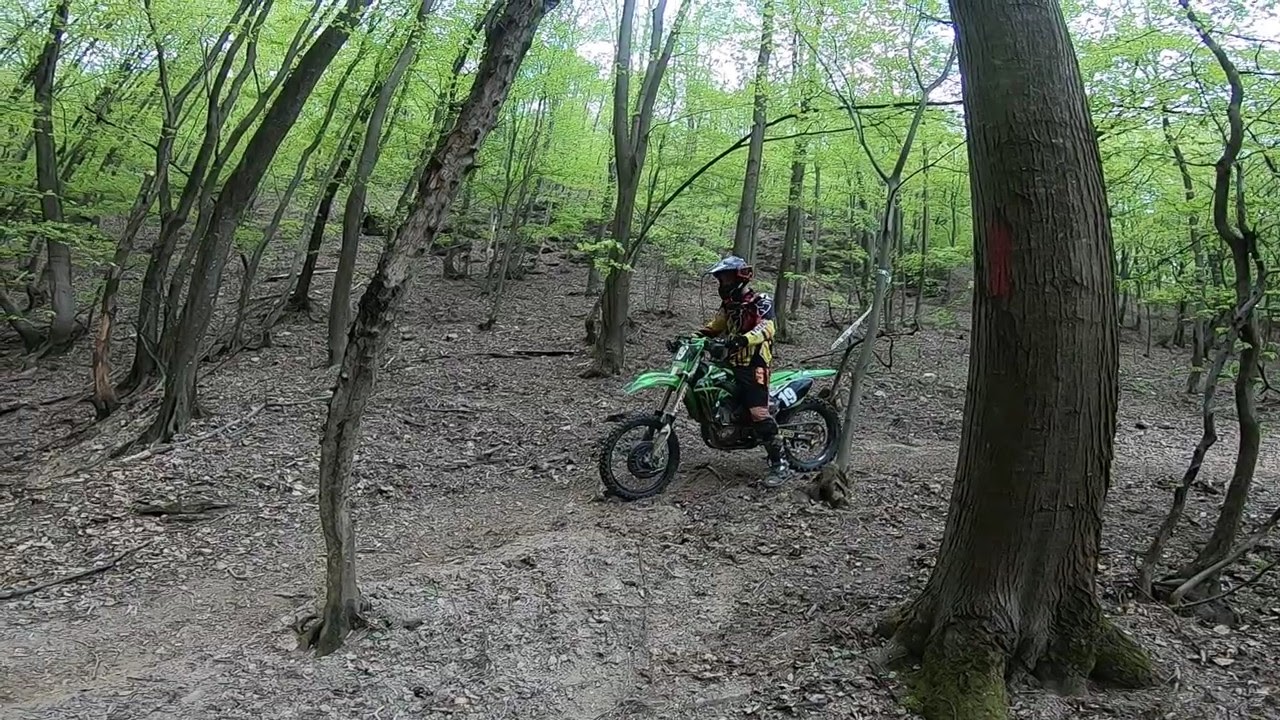In this image, a motorcyclist is navigating a dirt path through a unique forest. The forest features trunks of various trees that curve elegantly, creating a whimsical, almost parenthetical frame around the scene. The light filters through the loosely spaced canopy, revealing patches of sky on what appears to be a bright day. The forest floor is a mix of dirt and dried brown leaves, devoid of vegetation, lending an open, rugged feel to the trail.

The focal point of the image is a motorcyclist, centrally positioned, riding a green dirt bike with black tires and a black seat marked by the number 19. The rider is outfitted in black biking gear with yellow accents on the jacket and a black helmet featuring a dark visor. Despite being surrounded by a dense array of wavily and distinctively swayed trees, the trail itself is clearly defined, allowing the motorcyclist to ride smoothly.

In the background, vibrant green leaves provide a stark contrast to the bare forest floor. The overall composition suggests a dynamic movement through a naturally sculpted woodland path, with the curving trunks guiding the viewer's gaze towards the speeding motorcyclist.